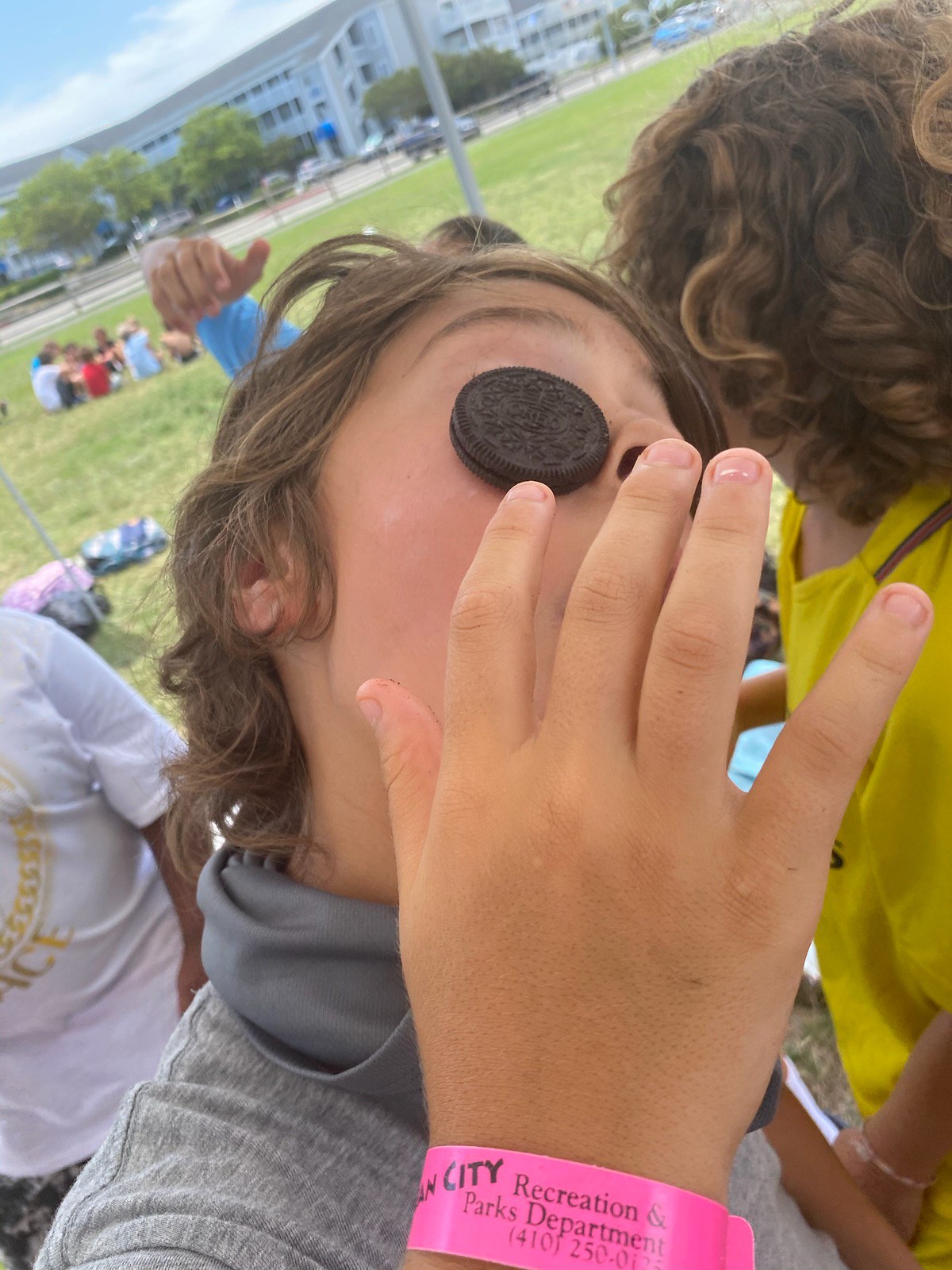In a lively park setting, young children and young adults are seen goofing around and enjoying their day. Central to the image is a person with shoulder-length, androgynous hair, striking a playful pose by balancing Oreo cookies over both eyes. They are partially obscuring their face with their hand, which sports a distinct pink wristband marked with "Recreation and Parks Department" and a phone number. This person is dressed in a gray shirt with a hood. Flanking this individual are two people, one in a yellow outfit on the right and another in white on the left. The group stands on lush green grass, with a background featuring seated individuals scattered throughout the park. The backdrop includes a road with light traffic, various trees, a large white building, parked vehicles, and a glimpse of sky in the top left corner. The colors in the scene range from gray and dark gray to vibrant hues of yellow, green, red, and light blue, highlighting the rich and diverse surroundings. The image captures a joyous, carefree moment in a public park in the middle of the day.